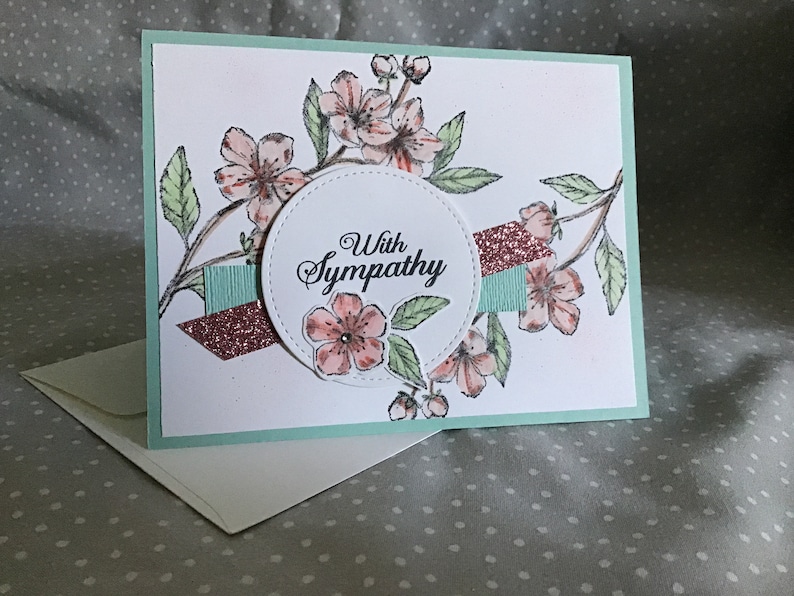This image depicts a close-up photograph of a sympathy card and its envelope, set against a light gray background adorned with white polka dots. The card, standing upright towards the top center of the image, features a horizontal design with a light green border framing a white inner section. It's embellished with floral motifs—red flowers with green leaves—flanking both sides of a central embroidered patch. This circular patch, slightly raised with stitching along its edges, bears the words "With Sympathy" in black text. Below the patch is an illustration of a red flower with two leaves, while similar flowers and stems appear above and to the sides. Positioned beneath the card is a white envelope with its top left corner and flap visible. The setting, suggested by the patterned fabric and the card's somber message, implies a context of mourning or a funeral.